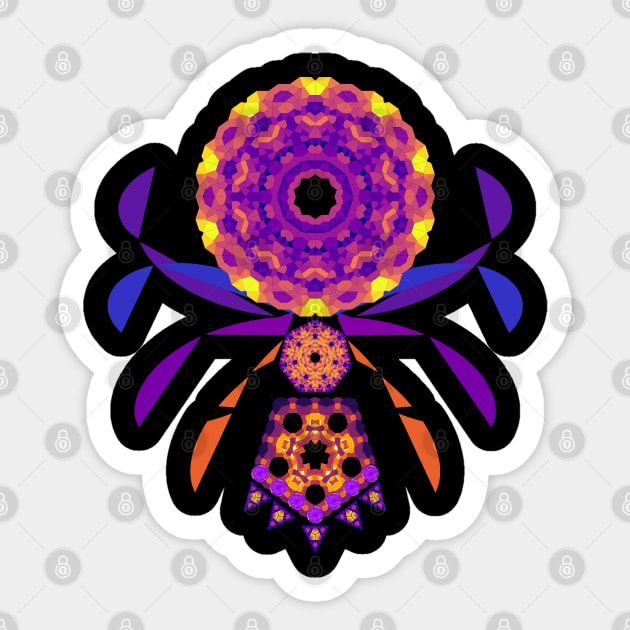This image features a digitally drawn, psychedelic logo or sticker set against a gray, watermark background adorned with lines, circles, and a diamond pattern, including locks to safeguard the design. The central figure resembles an artful, abstract spider or the back of a girl's head with an array of geometric patterns. At the top, there is an imperfect, flowery circle with a black center, extending with pink, blue, and purple hues towards the outer edges, highlighted by yellow dips. Blue and purple appendages flank the sides. The lower portion showcases a feather-like triangular extension blending purple, yellow, and orange colors. The entire figure is encapsulated by a prominent black outline, adding to its striking visual appeal.